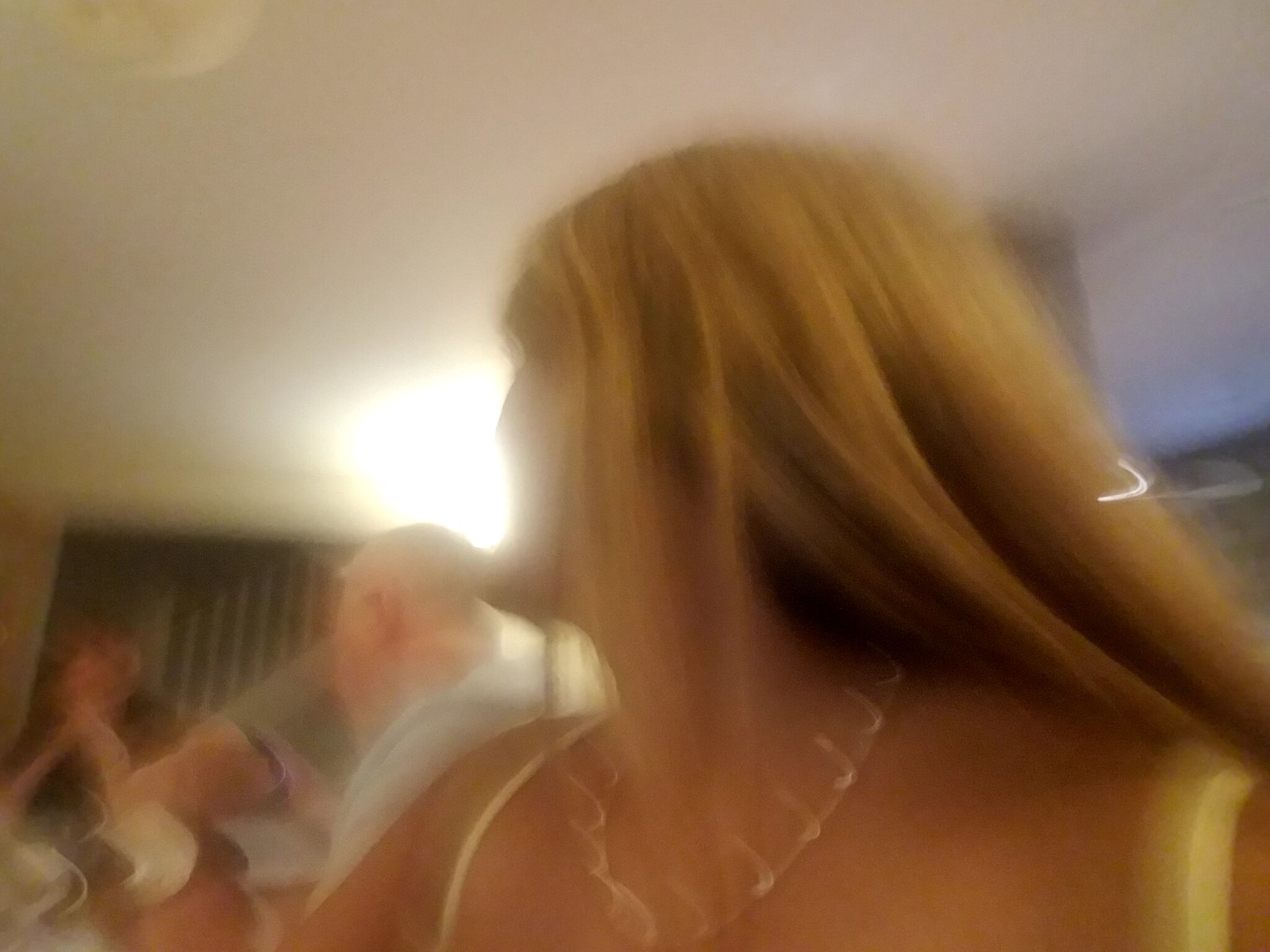In this color photograph, cloaked in a notable blur, we observe an intimately close shot of a lady with long, yellowy blonde hair featuring highlights. She wears a striking silver necklace adorned with loops and a distinctive dress with skinny straps, possibly in a yellow spandex wrap style. The ambient light in the room casts a gentle illumination on her face, heightening the sense of mystery and depth. The lady, partially captured in side profile, gazes back toward two men in the background. The first man, clad in a light-colored shirt, stands while seemingly engaged in conversation with another man seated at a table. This seated man has his hands thoughtfully crossed under his chin, resting on the table. The backdrop features green drapes and a ceiling illuminated by reflected light, suggesting an indoor setting, possibly a house. A gray structure with vertical lines, perhaps a support beam, adds a structural element to the scene. The overall ambiance hints at a social gathering, possibly a party.